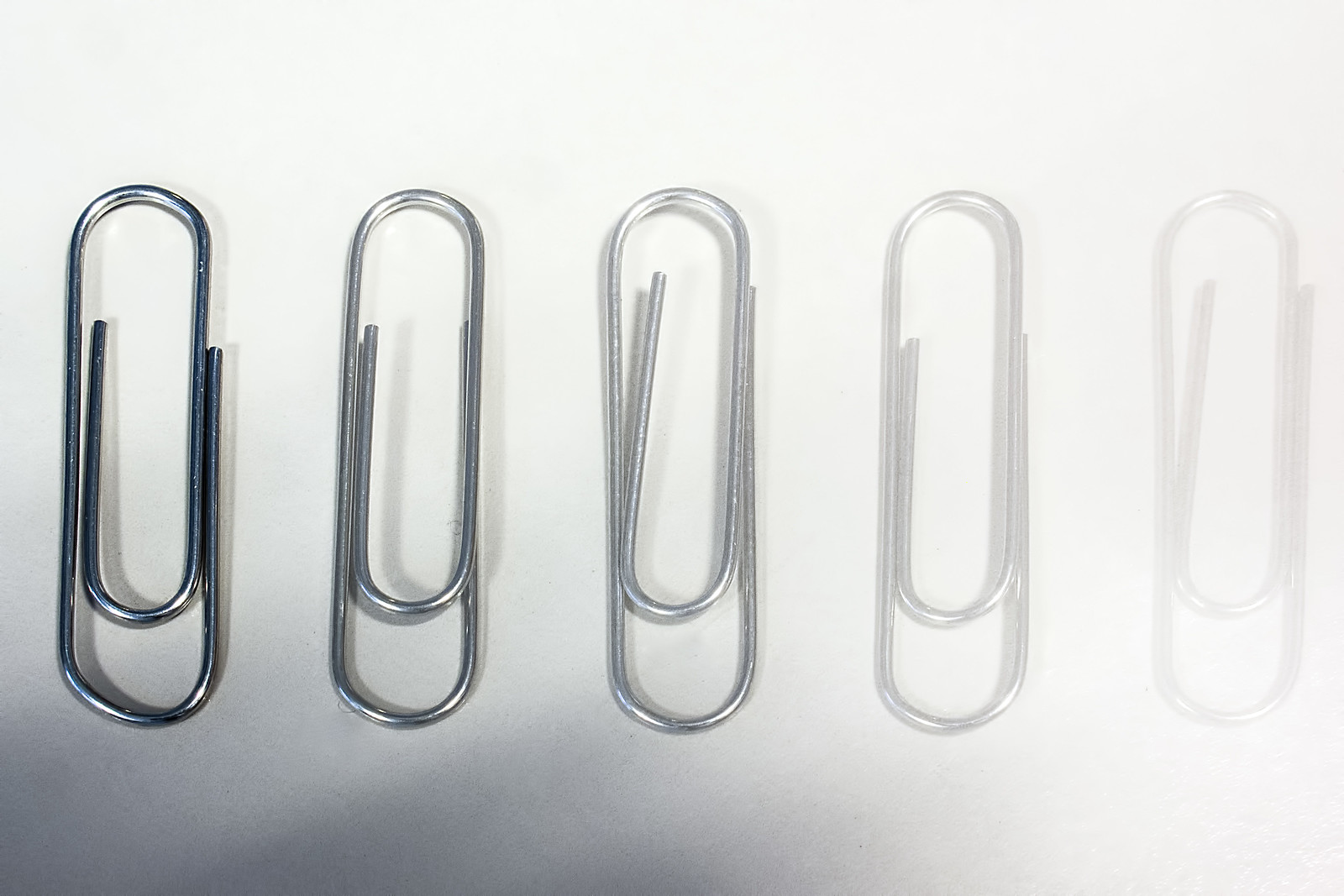The photograph depicts five paperclips arranged in a diagonal line against a white background. A slight shadow is visible in the bottom left-hand corner. The paperclips are sequenced from left to right, with each progressively becoming lighter and harder to see. The leftmost paperclip is a dark gray metal, catching the most light and appearing the clearest. Adjacent to it is a slightly lighter gray paperclip, followed by a third in a medium gray shade. The fourth paperclip is a pearl silver color, markedly lighter than the previous ones. Finally, the fifth paperclip on the far right is almost completely white, its outline barely distinguishable against the white background. Light casts across the image, intensifying the shadows on the left three clips, while the right two remain without shadows.